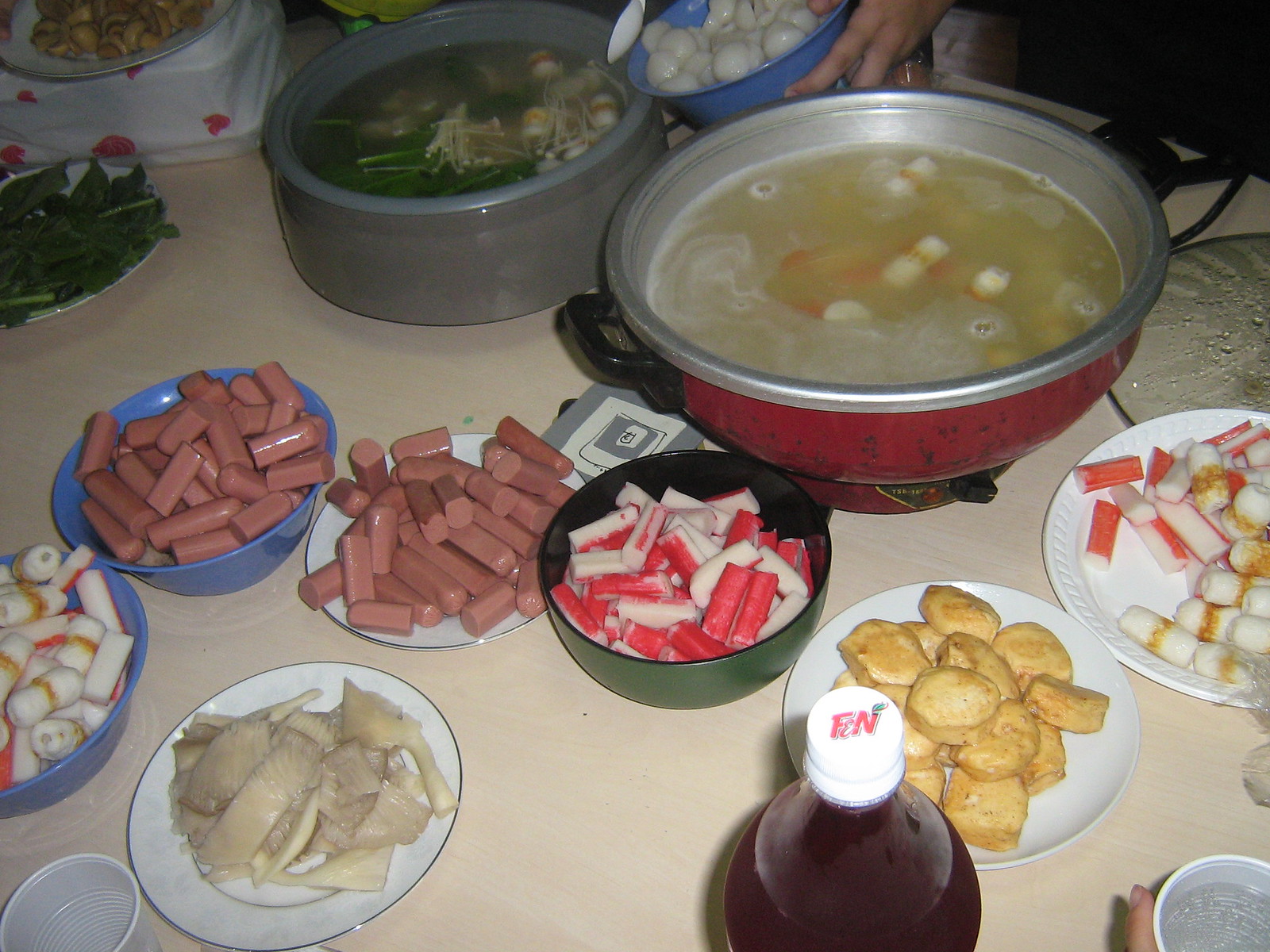The image showcases a diverse and home-style spread of various food items, laid out on a large white table that resembles a picnic setup. Central to the scene is a prominent red pot filled with some kind of liquid and food, possibly soup. A collection of plates and bowls surround the pot, displaying an assortment of ingredients and dishes. To the left, on a blue plate, are sliced hot dogs or cocktail weenies, while nearby on a white plate lies what appears to be fish or mock crab. Another white plate, to the right, holds more mock crab or crab sticks.

Further back, there's a silver cooking pot containing green vegetables, perhaps spinach, with another plate of green leafy vegetables nearby. Toward the top of the arrangement, a blue container can be spotted, possibly housing onions. At the front of the display is a bottle containing a brown liquid.

Interestingly, hands can be seen in the background, actively involved in preparing the food by adding ingredients to the green-filled pot. Despite the varied nature of the dishes, the setup remains casual and inviting, reminiscent of a family gathering or homemade buffet.